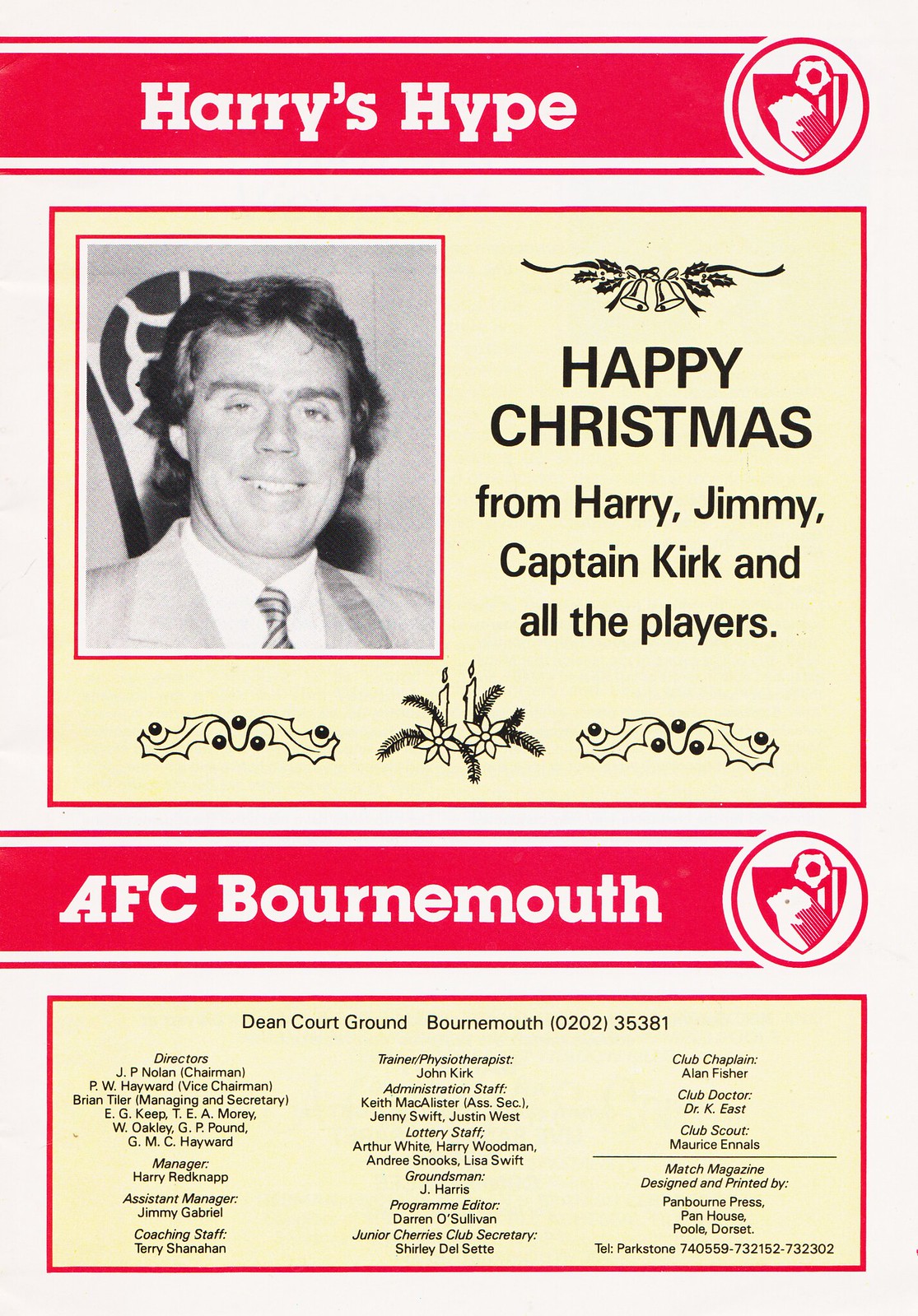This is an image of a vintage print advertisement from a magazine, likely a soccer club program for AFC Bournemouth. At the top of the page is a prominent red horizontal banner that reads "Harry's Hype" next to a circular shield logo. Below this is a horizontal, outlined box featuring a black-and-white photograph of a smiling gentleman in a suit and tie. The caption in this section says, "Happy Christmas from Harry, Jimmy, Captain Kirk, and all the players," embellished with holiday-themed line art, including holly and wreaths. Further down, another red banner features the AFC Bournemouth crest. Below this, a detailed list of the club's staff is provided, including the directors, manager, assistant manager, coaching staff, trainers, and the club doctor. The advertisement exudes a nostalgic, festive feel with its use of red and yellow spot colors on a black-and-white background, capturing the essence of a bygone era.